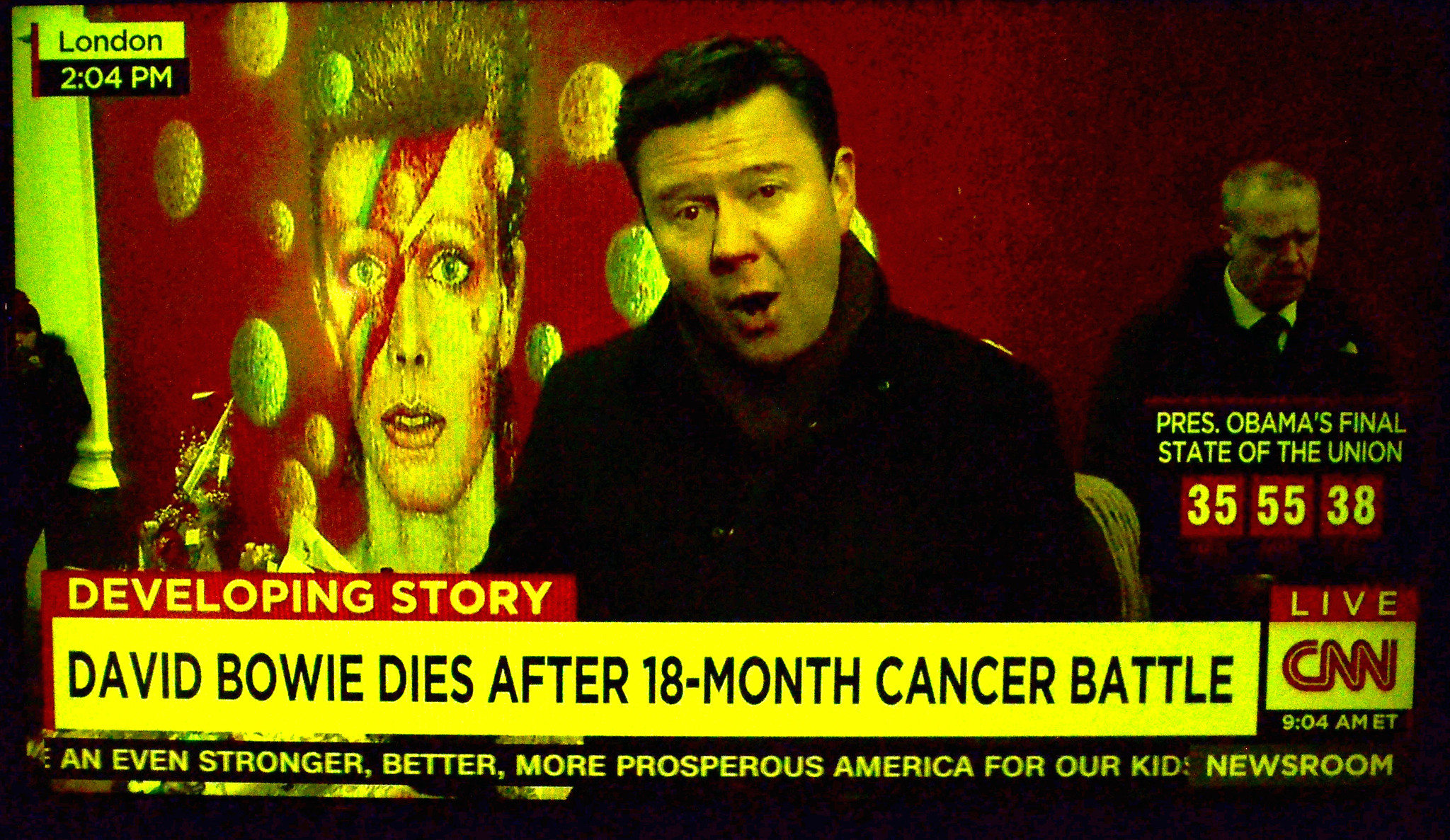This is a still image captured from a CNN news broadcast at 9:04 AM, featuring a segment on David Bowie's death. The screen displays several layers of information. At the bottom, there's a red rectangle with white text reading "Developing Story," and directly underneath, a white banner with blue and black text announces, "David Bowie dies after 18-month cancer battle." The broadcast is marked as "Live CNN" and "9:04 AM ET," with additional text mentioning "Prez Obama's final State of the Union, 35-55-38."

In the image, a news anchor with dark hair is seen speaking, wearing a black jacket and what appears to be a red scarf. To his right stands another man in a black suit with a black tie and a white shirt. Both figures are on the right side of the screen. On the left side, there is a prominent portrait of David Bowie featuring his iconic red lightning bolt makeup and pompadour hairstyle, with some background dots that add to the visual elements of the portrait. The overall lighting of the image is quite poor, suggesting it might have been a photograph taken from a TV screen. A slogan about "an even stronger, better, more prosperous America for our kids" is also visible, indicating broader news coverage themes. The image conveys a serious tone, focusing on the announcement of Bowie's death and upcoming national events.